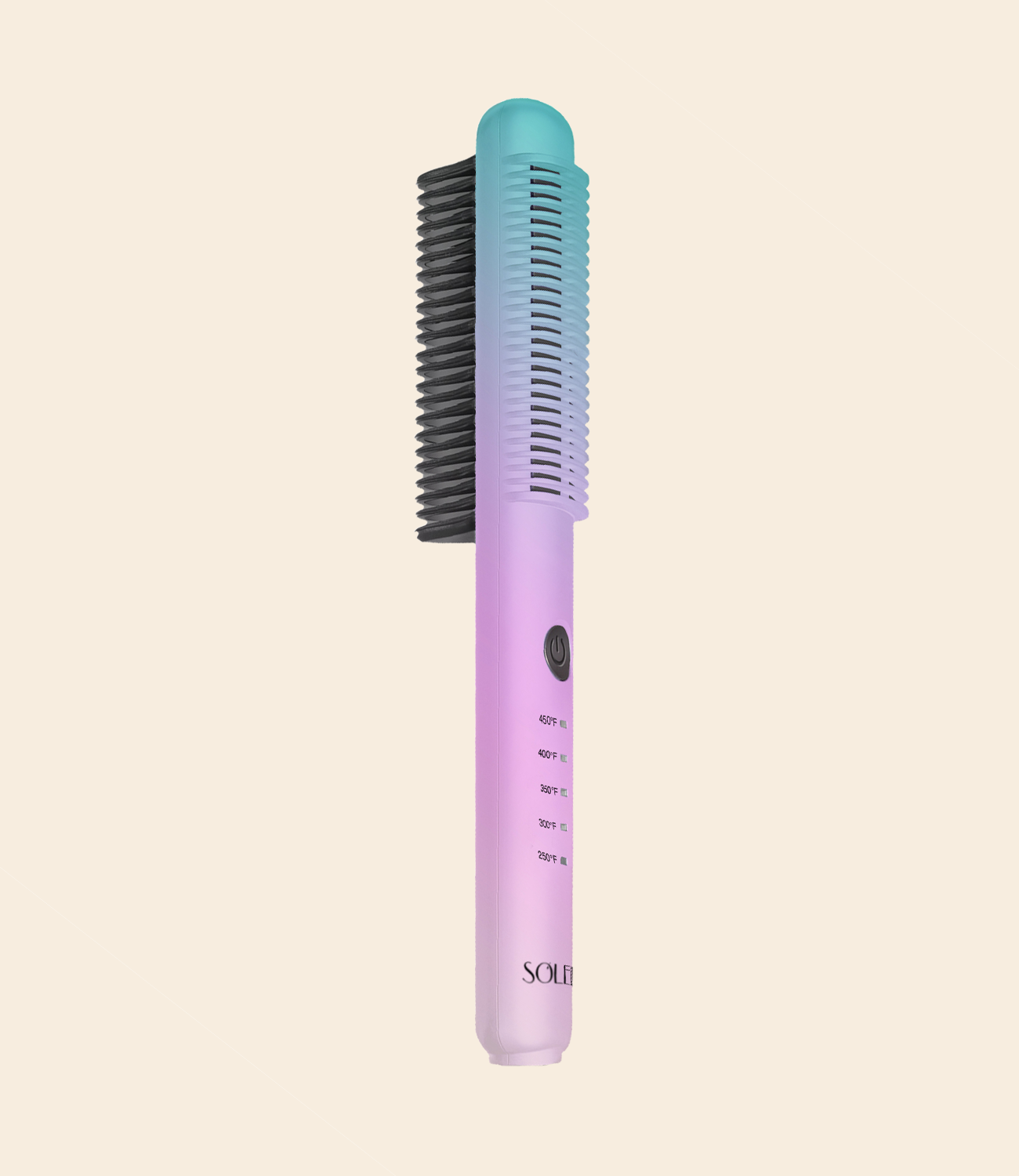The image depicts what appears to be an electric hairbrush, characterized by a smooth, gradient ombre color. The handle starts with a light purple at the base, transitions through various shades of purple and blue, reaching a turquoise or teal color at the top. A subtle transformation in color is evident, making the handle visually appealing. The bristles, positioned on the left side of the brush, are black and appear to be made of hard rubber. There is distinct black text on the handle reading "SOLAR" along with a series of temperature settings marked in Fahrenheit: 250, 300, 350, 400, and 450. A black power button is also present on the handle. This device is set against a soft pink background.